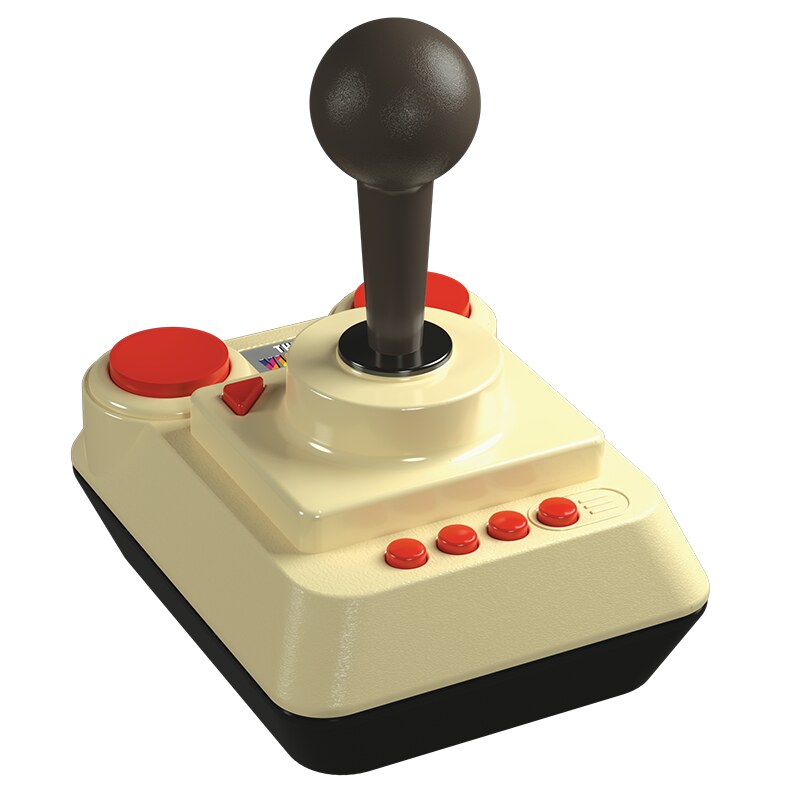The photograph showcases a vintage Atari joystick, predominantly in a beige or cream color with a contrasting black base. At the center, the black control stick protrudes, encased in a raised platform that emphasizes the cream-colored foundation. The joystick itself ends in a shiny spherical top, reflecting a subtle light source, suggesting a polished surface.

Positioned around the joystick are several distinct red buttons. In the front, there are four small circular red buttons, grouped together near the center. On the upper part of the joystick, two larger red circular buttons are found in each corner, giving it a balanced design. Additionally, there's a smaller triangular red button located on the upper left side of the platform, adding a unique geometric element to the controller.

Though the background of the image is plain white, which accentuates the joystick's colors and features, there is barely visible text or labeling on the backside of the joystick. This descriptive scene is set against a backdrop of gaming hardware aesthetics, capturing the essence of retro gaming equipment.